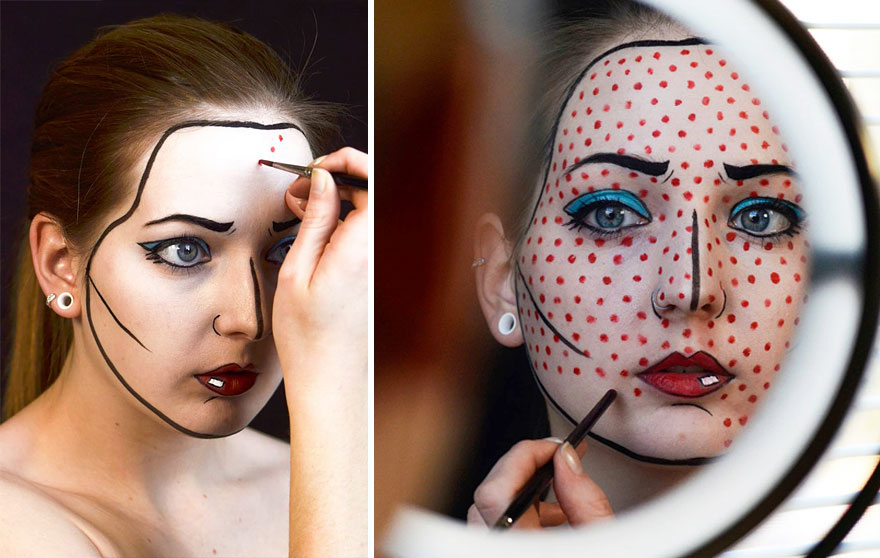The two side-by-side color photographs depict a young Caucasian woman with reddish, straight hair pulled back into a ponytail, meticulously applying elaborate face paint, possibly for a theatrical performance or costume event. In both images, she is seen mostly in right profile, focused intently as she looks into a makeup mirror. Her right ear bears two earrings: a small ear cuff and a plug stretching her earlobe.

The first photo shows the woman in an initial stage of her makeup application. She uses small paintbrushes to outline her face with a black line, creating a bold frame around her features. Her eyebrows are exaggeratedly drawn in black, and her eyes are adorned with blue eyeshadow, intensified by black outlines and long, thick eyelashes that extend into cat-eye wings. A striking black stripe runs down the center of her nose, accentuating the flares of her nostrils.

In the second, more developed phase shown in the right-side photo, the woman's progress is evident. The image captures her reflection in the round frame of the makeup mirror she uses. Her blue eyeshadow is more prominent, and she has added red polka dots symmetrically across her face, creating a grid-like pattern. Her lips are painted bright red, framed by a black outline, with a small white rectangle accentuating her lower lip. Her makeup evokes a vivid, cartoonish appearance, reminiscent of an elegant clown or a theatrical character.

These images vividly capture the transformation as the woman skillfully applies intricate and vibrant face paint, reflecting a blend of artistry and theatrical flair.